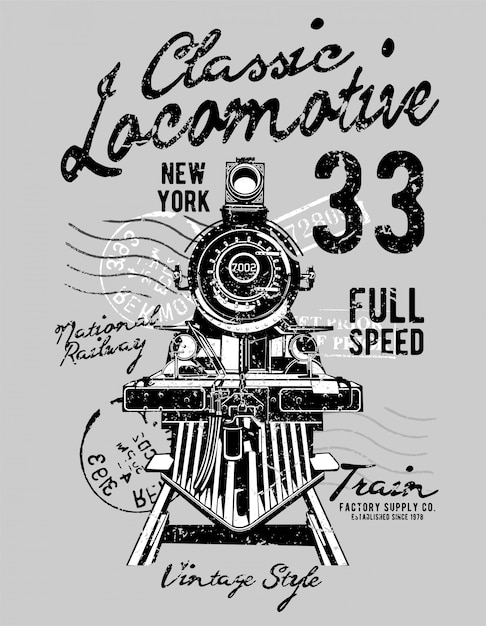This design features a black and white drawing of a vintage black steam engine train, numbered 7002, facing forward with a triangular cow catcher and a large lamp on top. The image is set against a light blue background, and the overall shape is rectangular, with the length twice that of the height. Surrounding the train are multiple lines of faded vintage-style text and stamp designs. At the top, in black script letters, it reads "Classic Locomotive." Beneath that, the text is split with "New York" on the left and "33" on the right. Additional phrases are scattered around the train, including "Full Speed," "National Railway," "Train Factory Supply Co.," and "Established since 1978." At the bottom, it says "Vintage Style" in script, completing the nostalgic feel of the image. The detailed artwork also shows the railroad tracks beneath the locomotive, emphasizing its readiness to race down the rails.